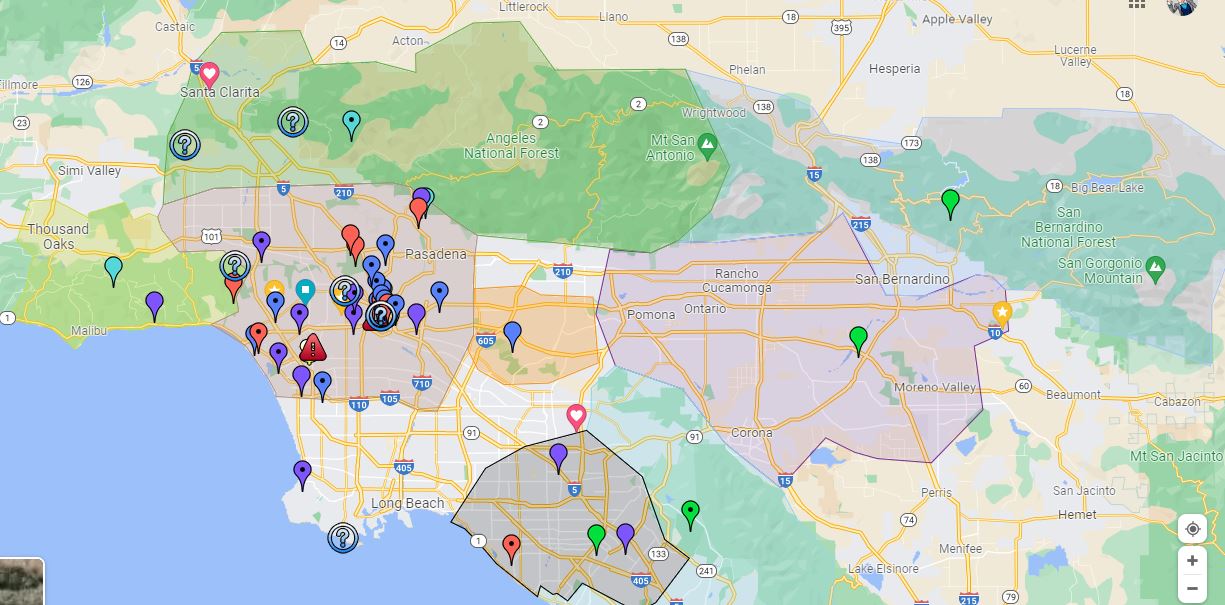This rectangular image, oriented with its long side running from left to right, appears to be a detailed screenshot from a GPS or map application focusing on Southern California. The map prominently features Los Angeles, Orange County, and extends to include parts of San Bernardino. Scattered across the map are various pins in multiple colors—green, purple, red, and turquoise, some with dots in their centers. A significant cluster of these pins is concentrated around the Glendale and Hollywood areas. Notably, there are also circles with question marks within this dense cluster and scattered in other regions such as Long Beach to the south and Santa Clarita to the north. Different zones on the map are indicated by slight variations in color shading, with areas like Orange County and San Bernardino distinctly demarcated.